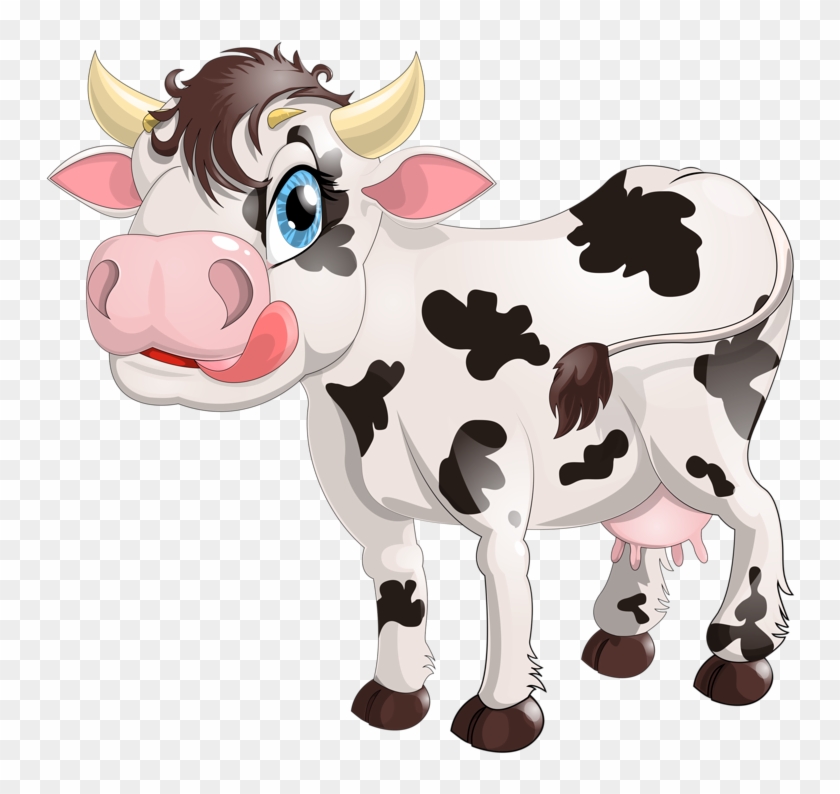This detailed illustration depicts a cartoonish black and white cow, set against a gray and white checkerboard background typical of PNG files. The cow, slightly off-center towards the right, displays a whimsical design with exaggerated features. It sports two prominent yellow horns and a tuft of brown hair atop its head. The cow's facial expression is highlighted by its large, blue left eye framed with yellow eyebrows and a sparkly black pupil. It has a pink snout complete with two nostrils, and its pink tongue is extended to the left, giving the impression that it's licking its chops. The inside of the cow's ears is also pink, complementing the color of its snout and udders. The cow's body is predominantly white adorned with randomly placed black spots, while its hooves and the tip of its tail feature a brown hue. This quirky, well-drawn cartoon cow straddles the line between realistic animal traits and playful, exaggerated proportions, making it an eye-catching element in the image.